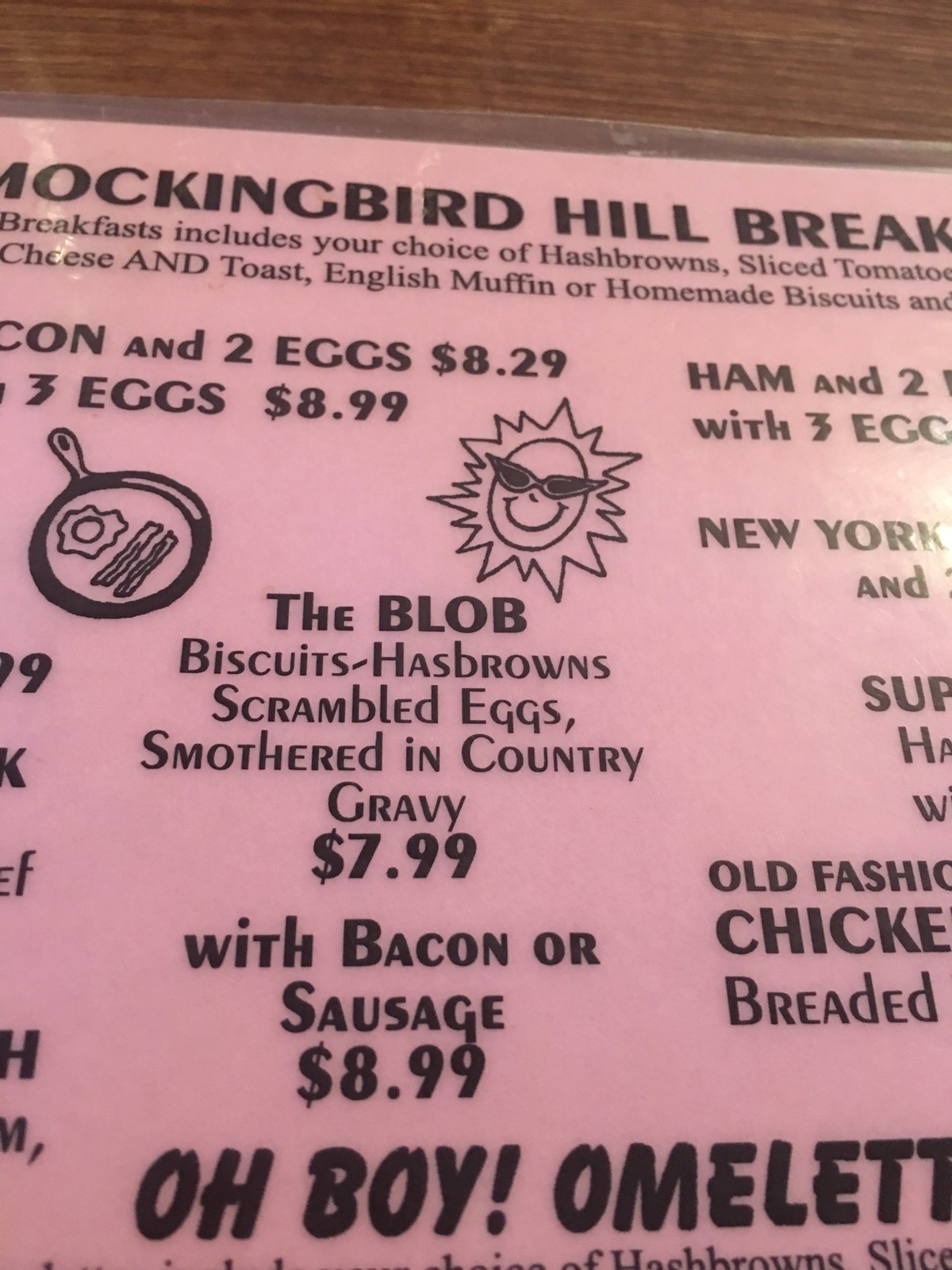A menu portion from a restaurant sits on a wooden table, bathed in a soft pink hue with a slight hint of orange. The menu's background is light, contrasting with the black text and illustrations. An artistic depiction of a frying pan containing bacon and eggs is featured alongside a cheerful sun wearing sunglasses. The menu title reads "Mockingbird Hill Breck," suggesting a breakfast-themed selection. 

One of the menu items includes breakfast dishes with choices such as hash browns, sliced tomatoes, cheese, toast, English muffins, or homemade biscuits. Priced at $8.29, a meal with bacon and two eggs is highlighted. Another dish, humorously named "The Blob," consists of biscuits and hash browns topped with scrambled eggs and smothered in country gravy, priced at $7.99, with the option to add bacon or sausage for an additional dollar. Among the menu’s offerings, a New York strip steak and a traditional (likely fried) chicken steak are mentioned, though parts of the text are cut off. At the bottom, the menu concludes with "Oh Boy Omelet."